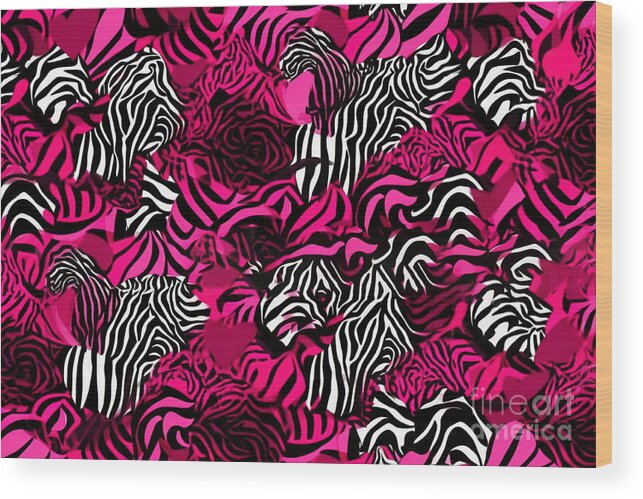This angled image captures an abstract, trippy painting on a canvas frame. The artwork features a striking, eye-catching collage of zebra stripe patterns in dark pink, white, and black. Interspersed with these traditional black and white stripes are patches of lighter pink and plum purple hues, creating a mesmerizing patchwork of colors and shapes. The painting's randomness and lack of a coherent form evoke a Rorschach-like effect, where prolonged observation reveals various interpretations, such as some swirls taking on the appearance of roses. The painting is printed on a wooden block, displaying the exposed grain along the right side. In the bottom right corner, there is a watermark in a transparent light gray font that reads "Fine Art America," adding a subtle signature to this vibrant piece.